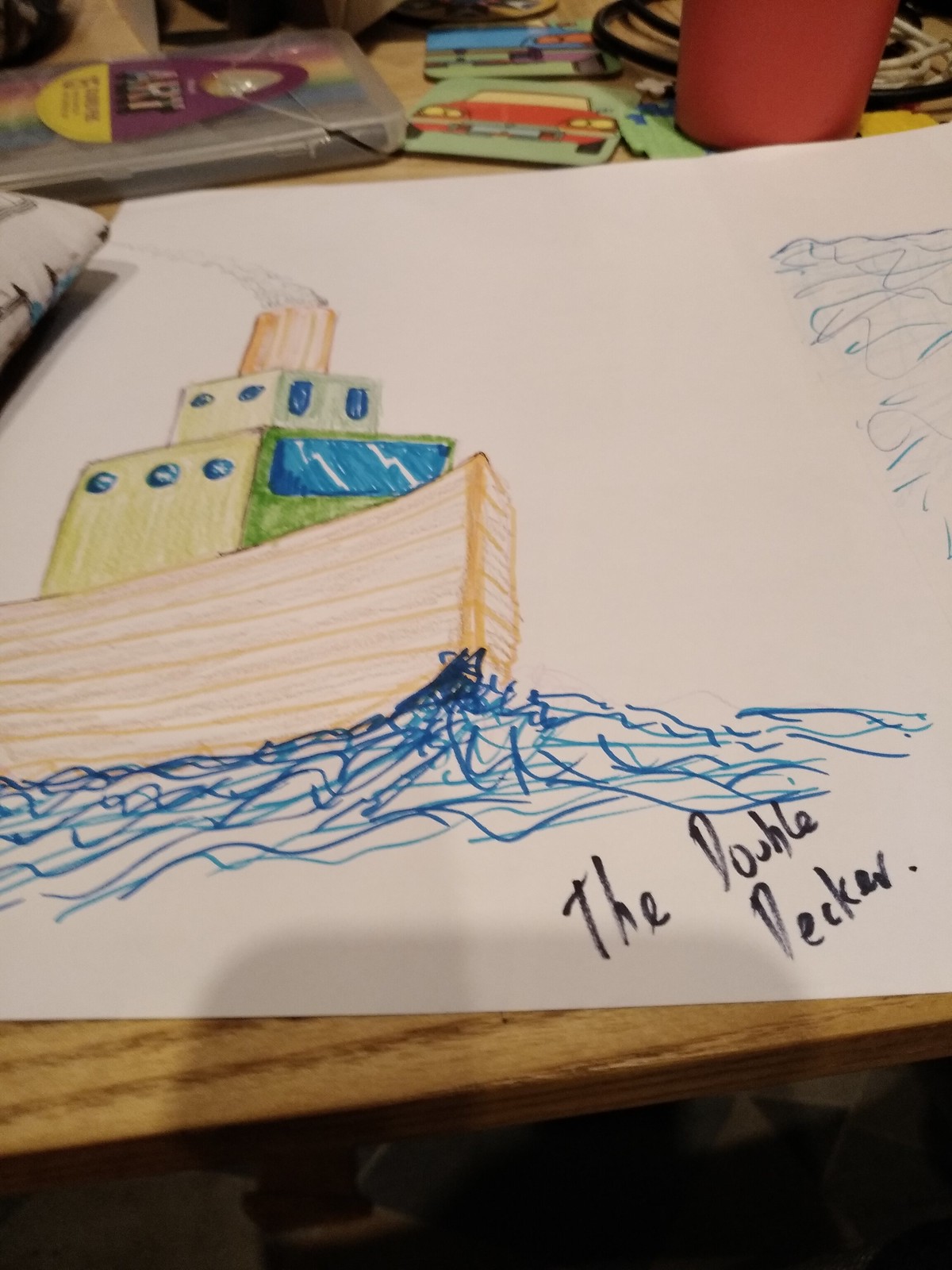This detailed image depicts a hand-drawn small-sized steamboat titled "The Double-Decker." The boat has a distinctive light brown base, resembling wood, crafted with colored pencils. Its two green, square-shaped decks, the top one being smaller and adorned with small blue portholes, sit atop the base, giving it its double-decker name. A light brown chimney or smokestack, emitting steam, crowns the vessel.

The scene is set against a blue sea, illustrated with blue felt-tip pen scribbles, on a white piece of paper resting on a brown table. The bottom right corner of the paper features the title "The Double-Decker" in black. Surrounding the drawing are various art supplies: on the top left, a plastic container holds colored pencils, beside which is a green piece with a drawn red card; a red cup sits to the right, adjacent to another green sheet of paper. Further right, a coiled white cable lies near the paper's edge. The boat faces right, stretching from just above the bottom of the canvas to the top.